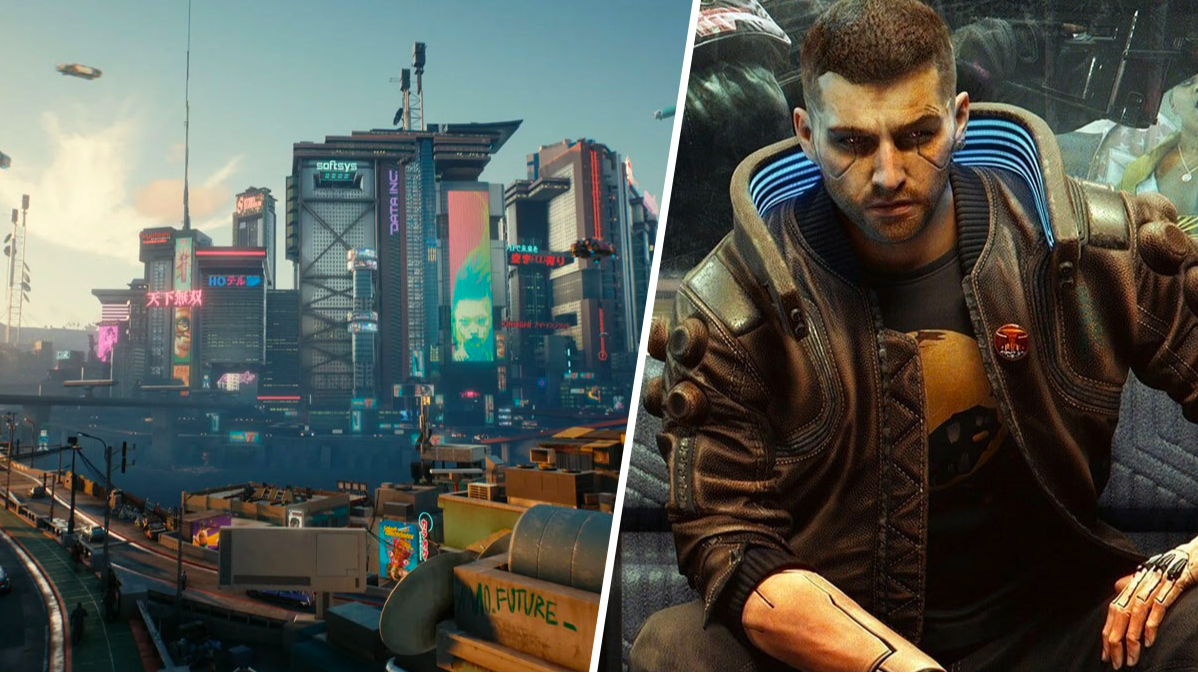The image is a detailed scene from a video game, presented as two rectangular panels divided by a diagonal white line. The left side of the panel depicts a dystopian, futuristic cityscape filled with colorful gray skyscrapers, industrial high-rise buildings, and large display neon billboards advertising various goods. The air appears dusky, creating a cyberpunk atmosphere. A plane and other spacecraft can be seen flying in the background. The city is alive with a bustling highway featuring multiple exits, numerous trucks, heavy traffic, and a bridge, adding depth and complexity to the urban environment.

On the right side of the panel is a rugged, young man who appears to be a game character. He has short hair and his eyes are marked with two prominent scars or streaks. Wearing a large leather jacket with a distinctive large collar, possibly wooden or futuristic material with lights embedded, he exudes a somber and contemplative demeanor as he looks downward. His sleeves are pushed up, exposing his forearms and hands which display tattoos and possibly electrodes. The man, who might also be a cyborg, is seated or kneeling near some tires, enhancing the gritty aesthetic with details like a red button or patch on his jacket and additional bumps on the fabric. The scene encapsulates the essence of a stylized, immersive video game environment.